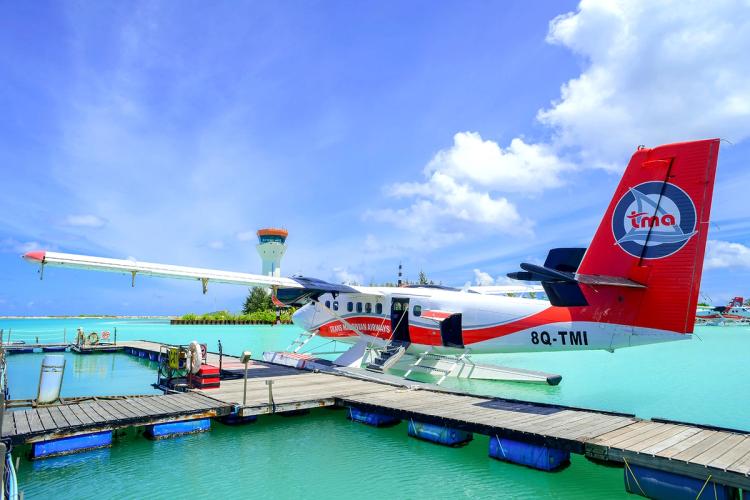The photograph captures a serene, tropical scene featuring a seaplane docked next to a wooden pier in crystal-clear, turquoise-green waters. The small aircraft, prominently white with a striking red wavy stripe along its side, has red accents on the tail wing and upper wing. The red tail fin bears the logo "TMA" in blue and white, along with the registration "8Q-TMI." The plane is equipped with boat-like appendages for water landings and has its door open, possibly awaiting passengers. The pier, lined with blue floating buoys, extends into the vivid, sunny day beneath a bright blue sky dotted with a few clouds. In the background, an air traffic control tower stands on a strip of land adorned with greenery, suggesting a well-equipped, inviting tropical destination perfect for an upbeat vacation.